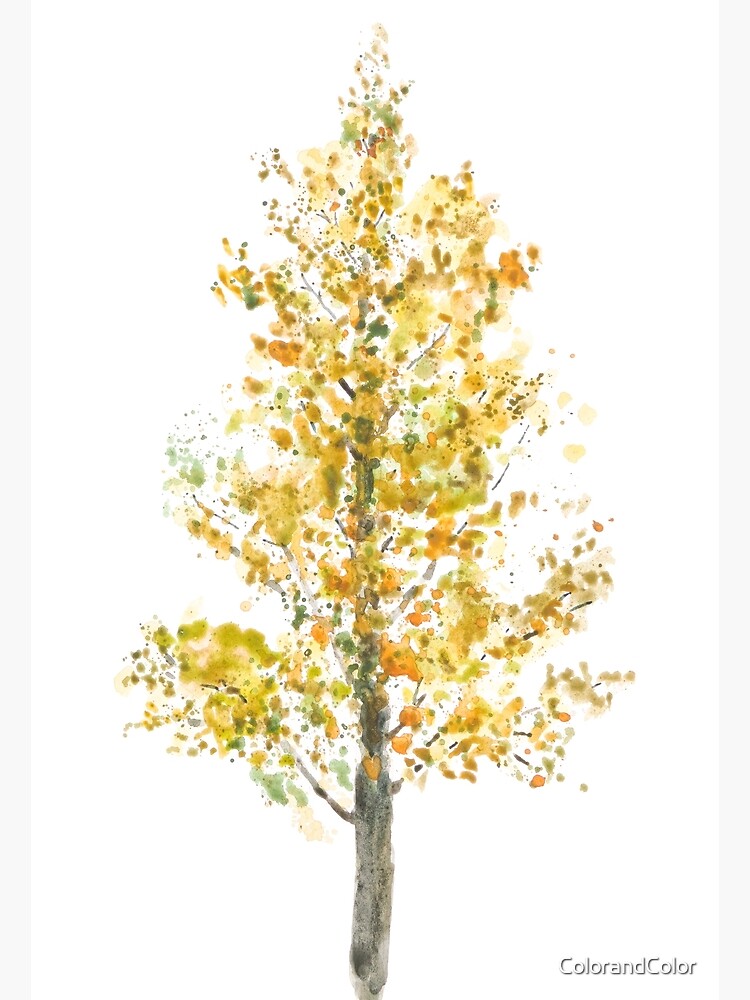The image is a beautiful, minimalistic watercolor painting of a tree set against a white background. The tree, centrally positioned, features a dark grayish bark and numerous wispy branches extending from a full base to a narrower top. Its leaves are predominantly yellow, with hints of light green, orange, and occasional dots of red, suggesting an autumnal scene. The leaves have been painted using a pointillism technique, giving a dotted, textured appearance. The overall effect is a simple yet vibrant depiction of a fall tree, capturing the seasonal transition from summer to autumn.